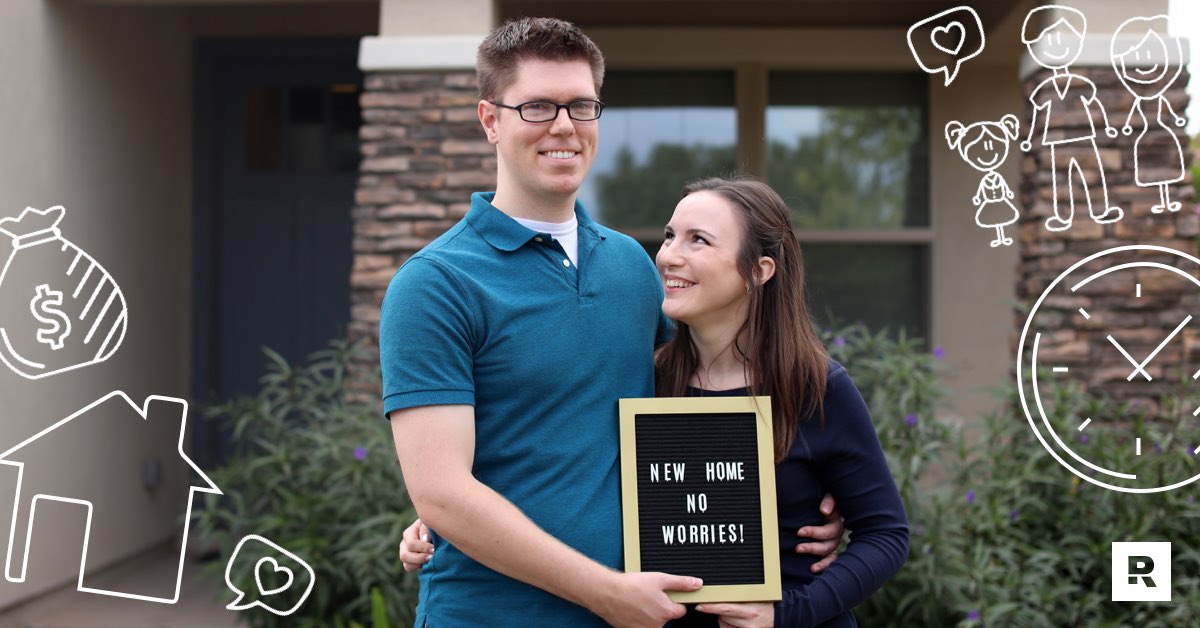In this image, a young couple, seemingly in their mid to late 20s, is posing in front of their newly purchased brick-fronted home. The man, positioned to the left, sports short, spiked brown hair with black-framed rectangular glasses, and wears a greenish-blue collared shirt with white buttons over a white t-shirt. Beside him, the woman, with shoulder-length brown hair, is smiling warmly up at him while her hand rests affectionately around his waist. She is dressed in a blue sweater. Both of them are holding a plaque that reads "New Home, No Worries". The backdrop of the image features a stone building with a four-pane window and a blue entry door. Overlaid on the image are various hand-drawn emblems, including a money bag, a house, and a heart. In the upper right-hand corner is an illustration of the couple with a young daughter standing beside them, suggesting a hopeful future. This joyful scene likely serves as a real estate advertisement.